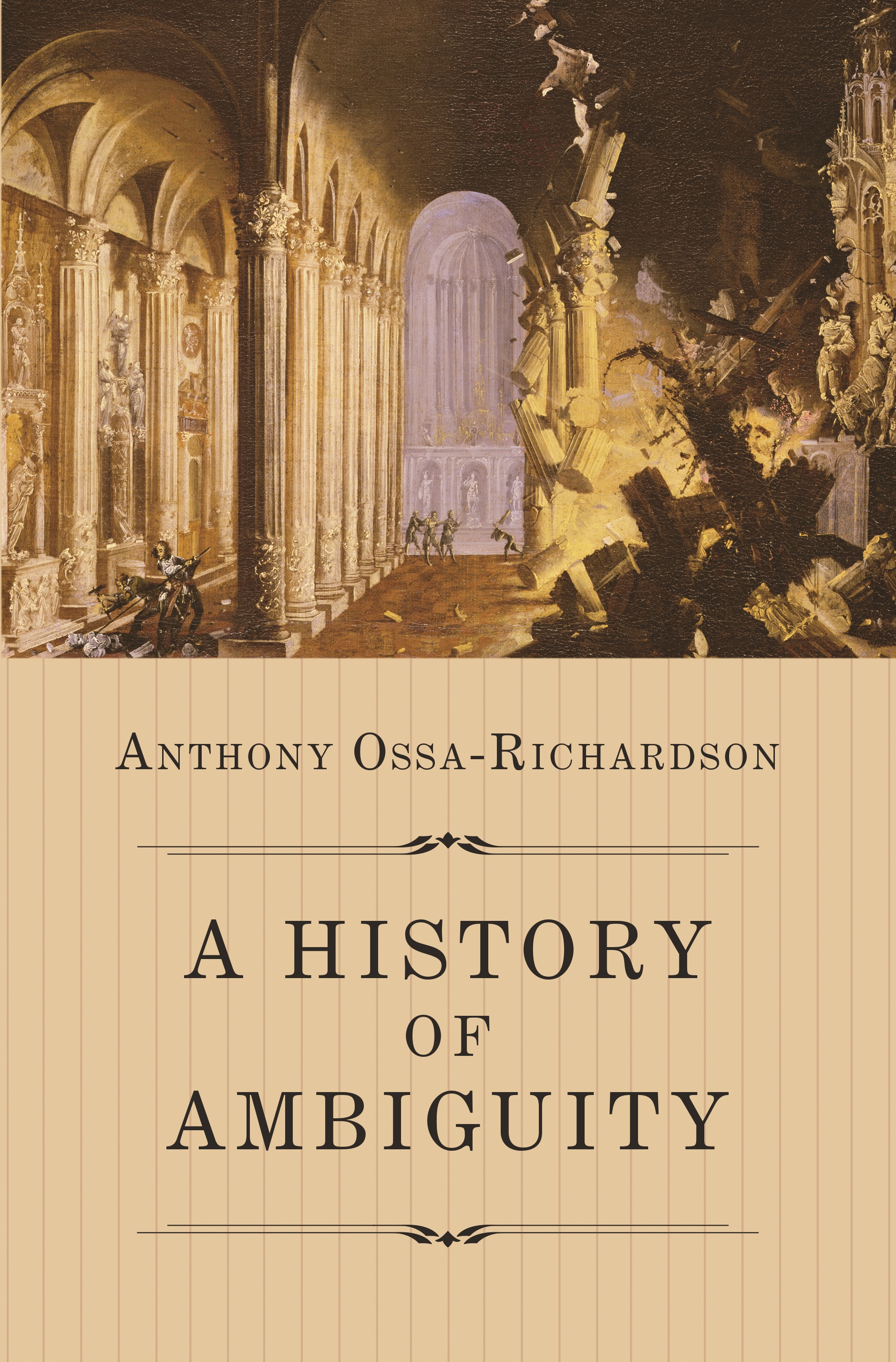The cover of the book, "A History of Ambiguity" by Anthony Osa-Richardson, features a richly detailed painting evocative of an ancient Roman or Greek temple. The top half of the image showcases a grand hall with tall, light tan columns and multiple archways receding into the background, giving a sense of depth and antiquity. At the far end of the hall, a series of statues, about five or six, can be seen; they appear to be Greek or Roman and suggest a once majestic structure now succumbing to decay. Some statues are crumbling, and there’s an indication of a battle scene with small, indistinct figures, possibly soldiers in ancient garb, amidst the ruins. The left side of the hall seems largely intact while the right side shows significant devastation, complete with falling debris. 

The bottom half of the book cover transitions to a light brown background with darker brown, vertically running lines. This section contains the book title and the author's name in dark text. The title, "A History of Ambiguity," is presented in a stacked format, neatly divided by horizontal design elements. The author's name, Anthony Osa-Richardson, is also prominently displayed, with "Osa-Richardson" hyphenated. The intricate and historical imagery combined with the striking textual design creates a compelling and thought-provoking cover.